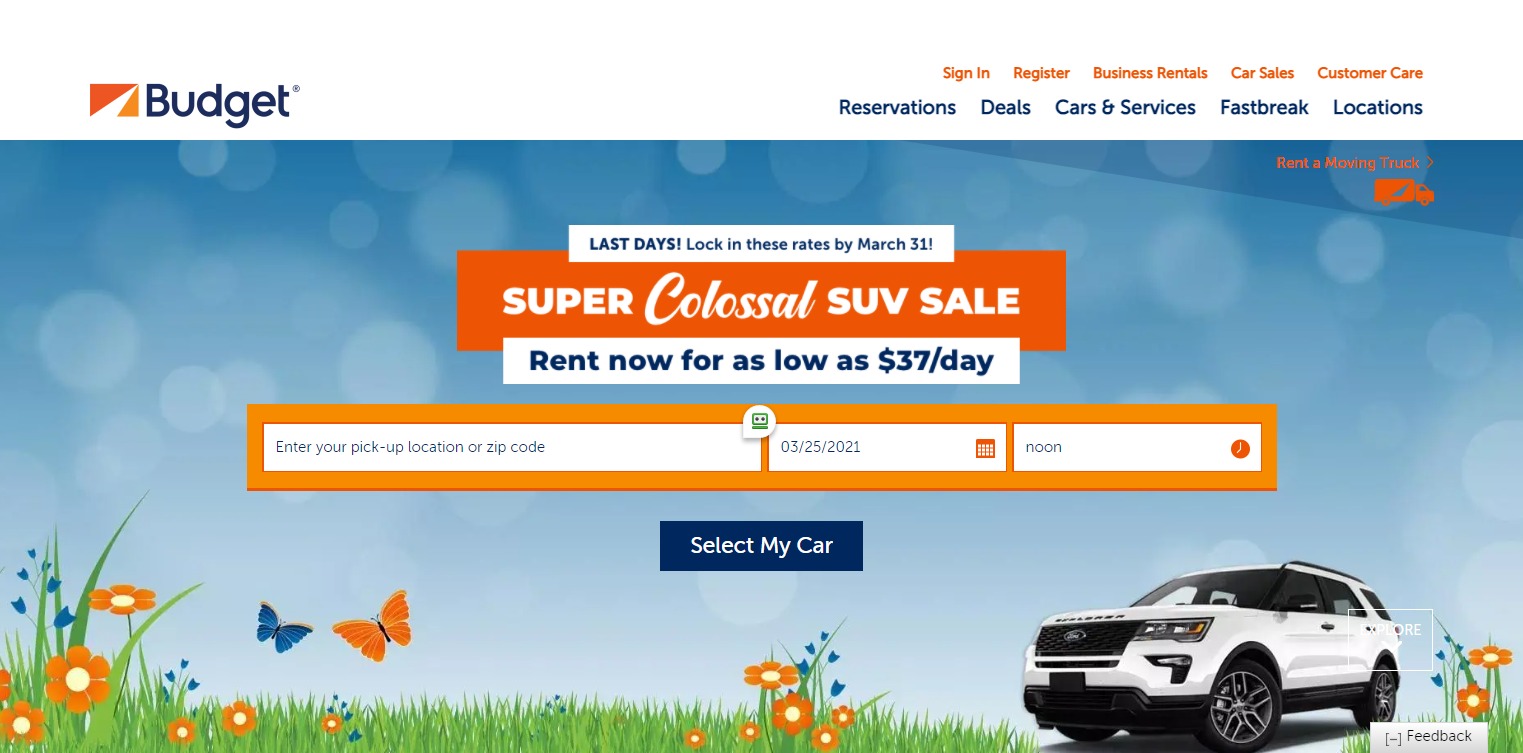Here is a cleaned-up, detailed caption for the image described:

---

The image is a screenshot from the Budget Car Rentals homepage. At the very top, there's a white border on the left side. Below, a vibrant, abstract design features a rectangular shape with bold colors: a red section starting from the bottom left corner angling up to the top right corner, transitioning into a white, road-like stripe that returns diagonally to the center. Surrounding this white stripe, the left section is red, while the right section is yellow. The 'Budget' logo is prominently displayed on the right side in large blue lettering.

In the center of the image, there's a navigation menu with small blue text featuring options: 'Reservations' (center), 'Sign In' (above), 'Deals' (below), 'Register' (above), 'Cars and Services' (below), 'Business Rentals' (above), 'Fastbreak' (to the right), 'Car Sales' (above), 'Locations' (below), and 'Customer Care' (above again). These menu items are placed in a stylistically colorful format with orange lines separating the sections.

Below this, a picturesque photo showcases a serene outdoor scene with a white car facing left. The backdrop features a blue sky with hints of green grass and orange flowers running across the bottom section, joined by orange and blue butterflies, creating a tranquil ambiance.

At the center of the image, a white tab contains blue text stating: "Last days to lock in these rates. March 31st." Adjacent to this, a large orange tab with bold white capitalized letters declares: "SUPER SUPER COLOSSAL SUV SALE." A smaller white segment underneath presents an offer in blue lettering reading: "Rent now for as low as $37 a day."

Immediately below are three interactive fields: the first allows users to pick their location, the second to select their rental dates, and the third field is for additional information. Concluding the form, a blue tab at the bottom with white text invites users to "Select My Car."

---

This caption provides a clear and detailed description of the homepage's layout and design elements.